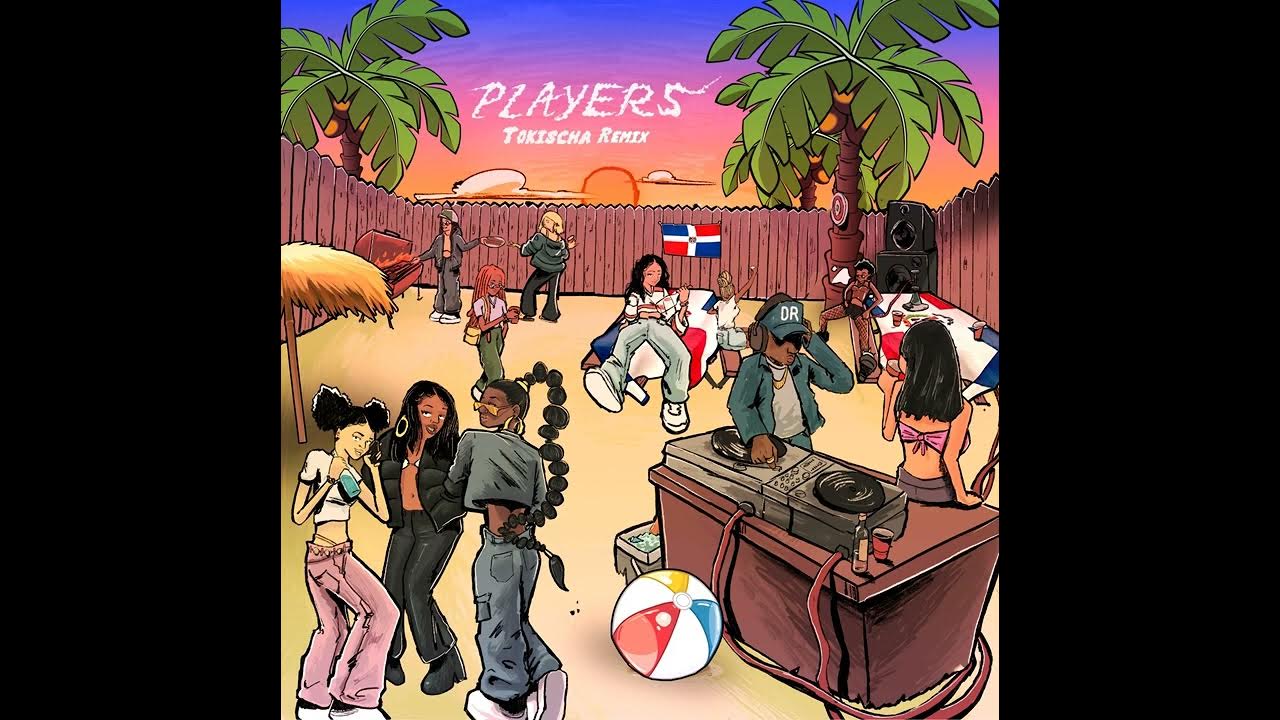This vibrant illustrated album cover, titled "Players: Tokisha Remix," captures the lively atmosphere of a backyard party set against a tropical, sunset backdrop. The enclosed party area, surrounded by a redwood plank fence with triangular tops, is adorned with three coconut palm trees—one within the yard and two just outside it. The fence encloses a sandy ground, enhancing the tropical vibe.

In the lower right corner, a DJ fiddles with his equipment on a table topped with a beach ball, while interacting with a woman seated on the same table. In the lower left, a group of women energetically dance together, contrasting with another woman who walks by someone barbecuing and handing out food nearby. Scattered throughout the middle of the scene are more partygoers dancing, socializing, and enjoying activities like smoking hookah at a table with a red, white, and blue flag featuring a white cross.

The sky is a breathtaking gradient from dark blue to pink and tangerine, highlighting the setting sun just above the fence. Adding a whimsical touch, text reading "Players Tokisha Remix" appears to be written in the clouds, emphasizing the album's title and creating a dreamy, festive atmosphere. The partygoers, dressed in urban clothing, animate this dynamic scene, where the sound of music, laughter, and the clinks of glasses bring this backyard bash to life.